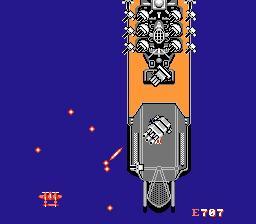This image appears to be a screenshot from a vintage video game, likely from the early Nintendo era, depicting a naval battle scenario from the Battle of Midway involving the Yamato battleship. Central to the image is a large, rectangular ship with an orange deck and a gray hull, representing a simplified battleship design. The ship is equipped with multiple gun turrets, including a prominent triple-barrel gun. The background is a simple dark royal blue, possibly representing the ocean. 

In the lower right corner, there is the label "E-707," with the "E" in purple and the "707" in white. The lower left corner features a double-engine aircraft. There are multiple small red dots and red streaks, indicating incoming fire directed at the ship. The red streak appears to be a projectile in motion, while dashed lines suggest other ongoing attacks. Amid the ship's details are additional smaller turrets. The simplistic and pixelated design of the ship, the minimalistic background, and the overall graphic style underscore its vintage nature.